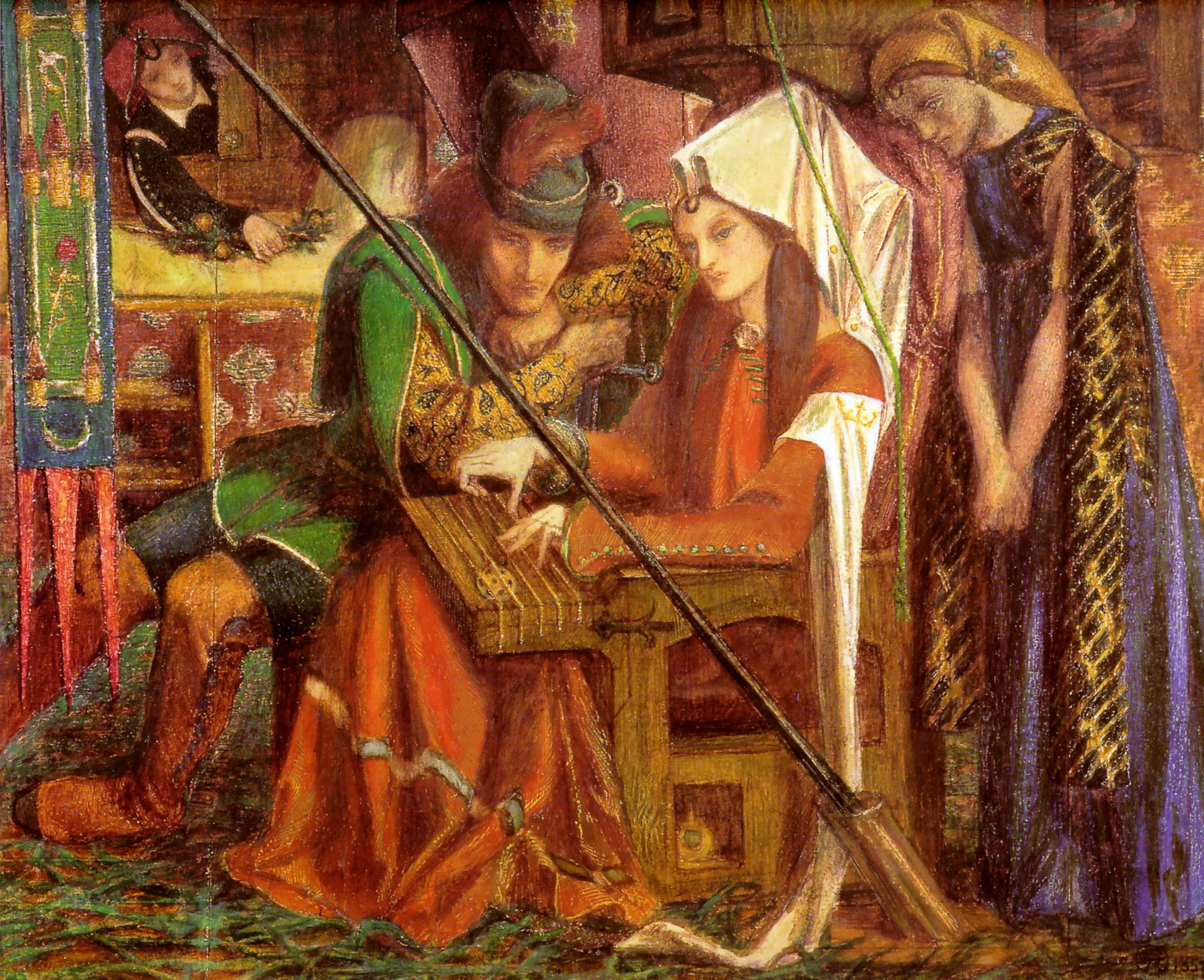The image depicts a historical painting set in what appears to be a courtly scene from the 1970s or 80s, emphasizing the attire and demeanor of its subjects. At the center, a woman clad in a rust-colored, floor-length dress adorned with silver rivets on her forearms and a brooch at her neckline sits on a large wooden chair. Attached to the chair is a musical instrument with five strings, which she is playing. She wears a white mantilla or similar renaissance headdress. Behind her, another woman in a blue draped dress stands with her hand resting on the back of the chair, leaning slightly forward. To the left, a man garbed in an ornate green jacket with a hat bearing a feather and brown boots leans on the arm of the chair, listening intently. Additionally, there is a black diagonal rod or staff mounted in front of the scene, and a flag is visible on the left side of the composition. In a window in the background, another man appears to be placing flowers on a countertop. The overall scene captures a blend of historical and musical elements, with each character contributing to the painting's rich narrative.